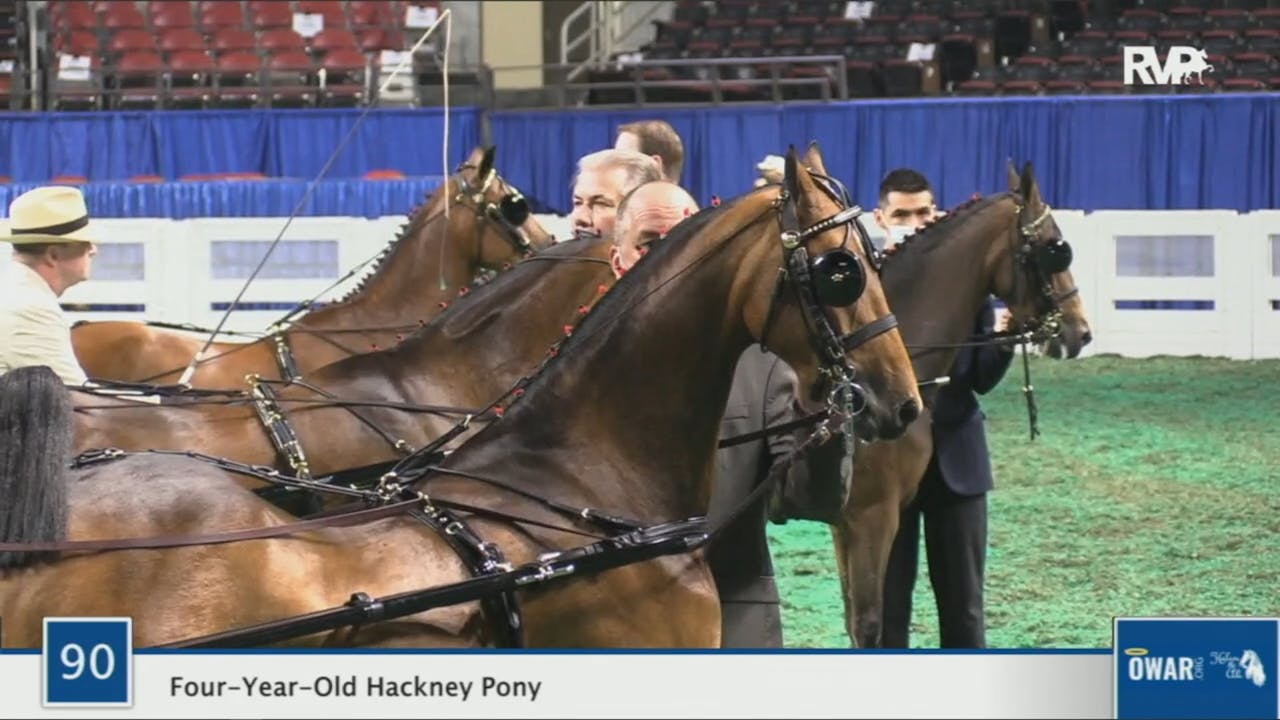Inside a grass-covered horse arena, a vibrant colored photograph captures an event involving four Hackney ponies. At the bottom left, the image is annotated with "number 90" and "4-year-old Hackney pony," suggesting the pony closest to the viewer is a 4-year-old. Each pony is adorned with blinders and traces, indicating they are either harnessed to a single wagon or perhaps preparing for a chariot-style race. The scene hints at the start of a race or show, with four men in front of the ponies, all dressed in formal suits, and one man donning a distinctive top hat, possibly serving as a judge. Adding to the dynamic moment, another person, positioned two horses away, holds a whip or crop.